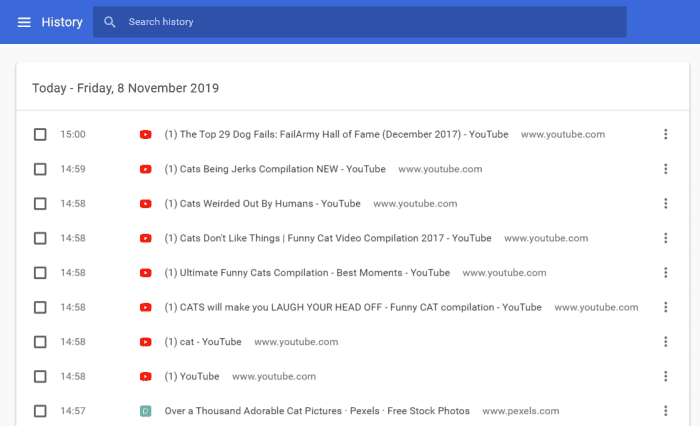Here's a detailed, cleaned-up caption for the image described:

The webpage features a predominantly white background with a blue border spanning the top inch of the page. On the left side of this blue border, three short horizontal white lines are stacked vertically, approximately half an inch long each. Directly to the left of these lines, the word "History" is displayed in white text. Adjacent to "History" is a long dark blue search bar extending almost to the right edge, with a white search icon and the words "Search History" in white within the bar.

Below the blue border, the top left corner of the page features the current date, styled as "Today - Friday, 8 November 2019." The left side of the webpage is lined with nine white boxes, each bordered in black. These boxes are associated with timestamps listed sequentially downward from 15:00 to 14:57:

- 15:00
- 14:59
- 14:58 (repeated six times)
- 14:57

To the right of the timestamps, the first seven entries display a blue or red YouTube play icon, while the bottom entry shows a blue square with a white circle inside. 

Further to the right, information about each video is provided, concluding with "www.youtube.com" for every entry. For example, the first entry is titled "The Top 29 Dog Fails, Fail Army, Hall of Fame, December 2017." Similar formats are used for each subsequent video listing.

On the far right border of the webpage, a column of three vertically aligned black dots is visible next to each entry, continuing down the page.